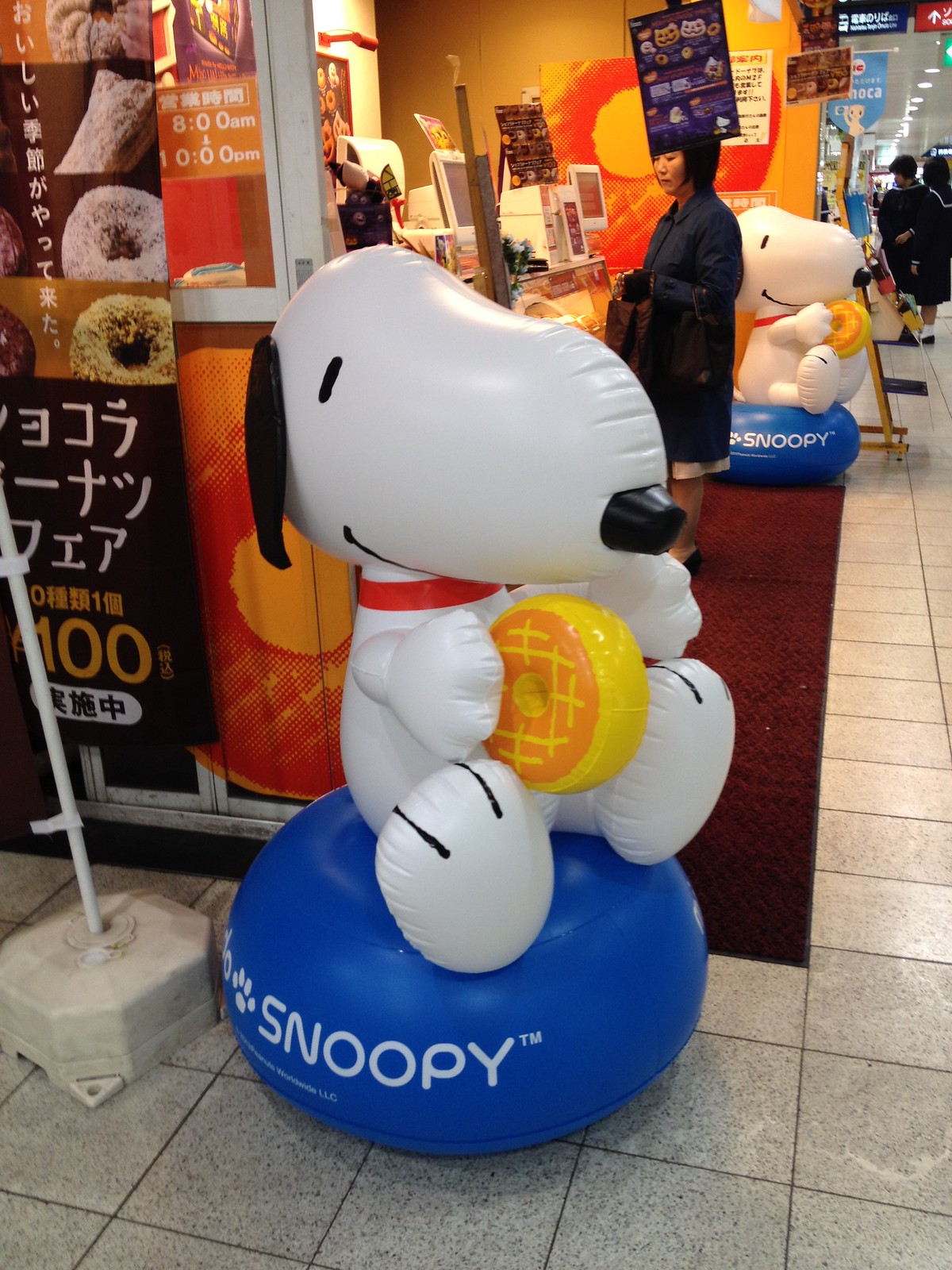This photo captures a vibrant scene likely set inside a mall, identifiable by the long hallway on the right side filled with people walking around, ceiling lights, and signs indicating buses and escalators. The focus is a colorful donut kiosk, predominantly orange and yellow, adorned with various donut images and prices, with signage written in Japanese. At the counter, a woman in a black jacket appears to be deciding on her order from a glass display of donuts.

Dominating the foreground are two inflatable Snoopy figures from the Peanuts comic strip. The Snoopy nearest to the camera is seated on a big blue donut emblazoned with the word "Snoopy" and paw prints, holding a smaller yellow donut. The second Snoopy, identical in appearance, is located on the opposite side of the kiosk, also holding a brightly colored donut. The entire scene exudes a playful and lively atmosphere typical of a bustling mall food court.